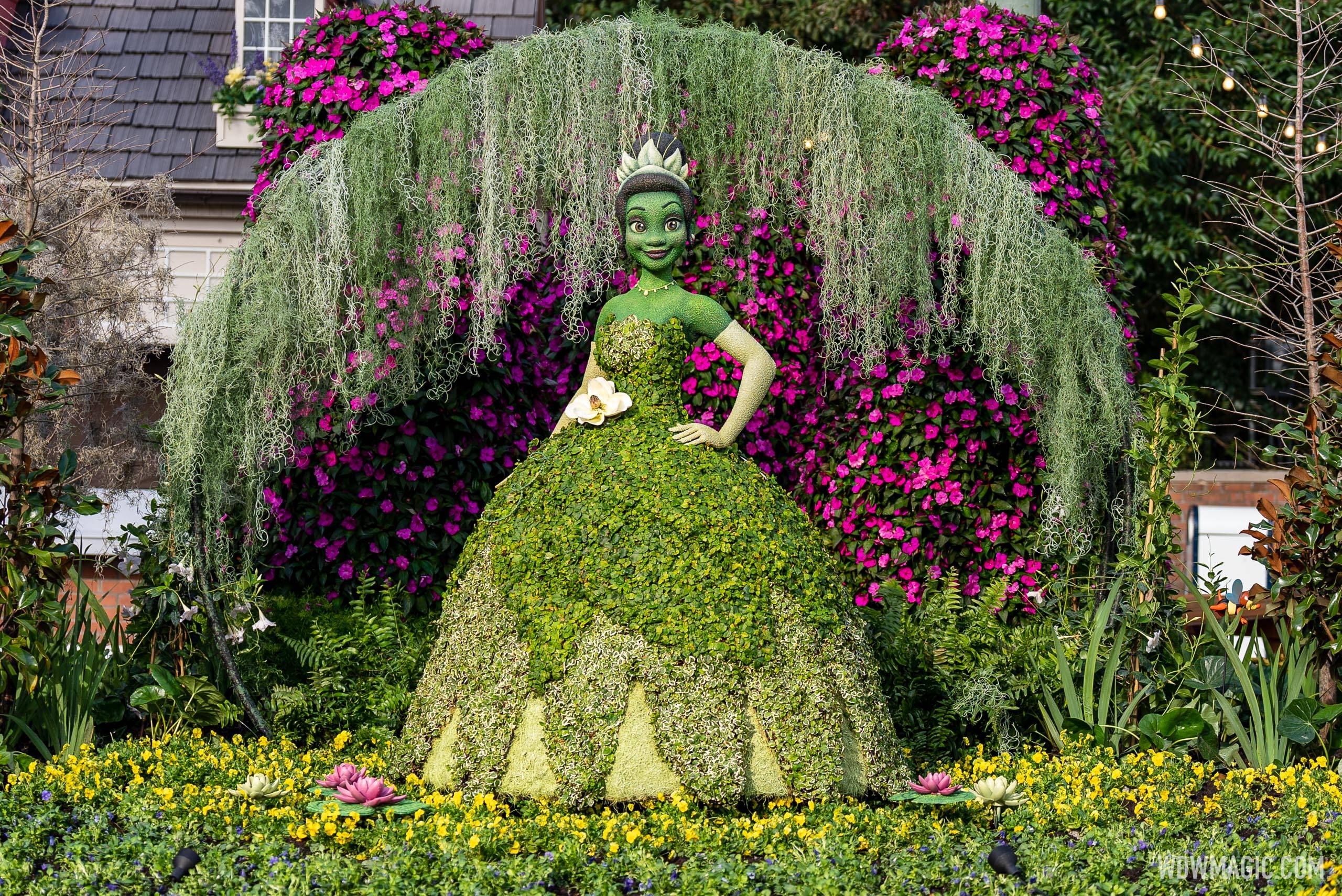The image portrays a meticulously crafted topiary of Princess Tiana from "The Princess and the Frog," located at the Walt Disney World parks. The figure is constructed using a metal framework filled with moss and adorned with diverse plants. Princess Tiana stands elegantly in a gown composed of various shades of green foliage, with distinct cream-colored flowers representing her gloves. Her green skin and purple eyes, likely derived from plant pigments, add lifelike details to the figure. A crown made of leaves sits atop her head, while a striking white flower adorns her hip. Her dress, comprising leaves and floral elements, demonstrates an artistic blend of different plants to replicate the character's essence without her traditional colors. She is positioned amidst a vibrant scene featuring numerous purple flowers, yellow blossoms at her feet, and an archway backdrop festooned with a mix of purple and pink flowers, some hanging moss, and additional bushes and trees. The entire display, possibly situated near a ride or restaurant, serves as a focal point for visitors. A discreet watermark, "wdwmagic.com," appears in the bottom right corner, hinting at the source of the image.